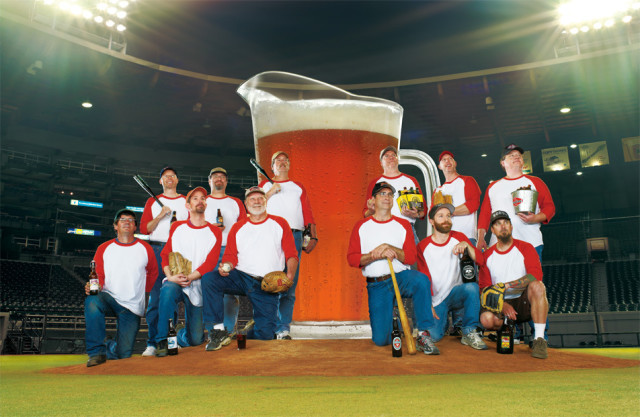The photograph captures a group of 12 men, presumably an amateur baseball team, posing spiritedly on a professional-looking pitcher's mound. The background displays an empty stadium with blue plastic seats and white spotlights illuminating the field from the upper corners. The team members are uniformly dressed in white baseball shirts with red sleeves, blue jeans, and baseball caps, except for one individual in the bottom right who is wearing shorts. They are arranged in two rows; the front row is kneeling or squatting on the brown dirt of the mound, while the back row stands.

Dominating the scene is a massive, clear glass pitcher of golden beer with a frothy white head, towering above the men. The green grass around the mound adds a vivid contrast to the predominantly white and red attire of the team. Many of the men are clutching beer bottles, with one on the right holding a metal bucket filled with beers and another holding a yellow carton of six beer bottles. Others are equipped with baseball gloves and black bats, positioned over their shoulders. The camaraderie and blend of sports and celebration are palpable, making for a lively and memorable image.